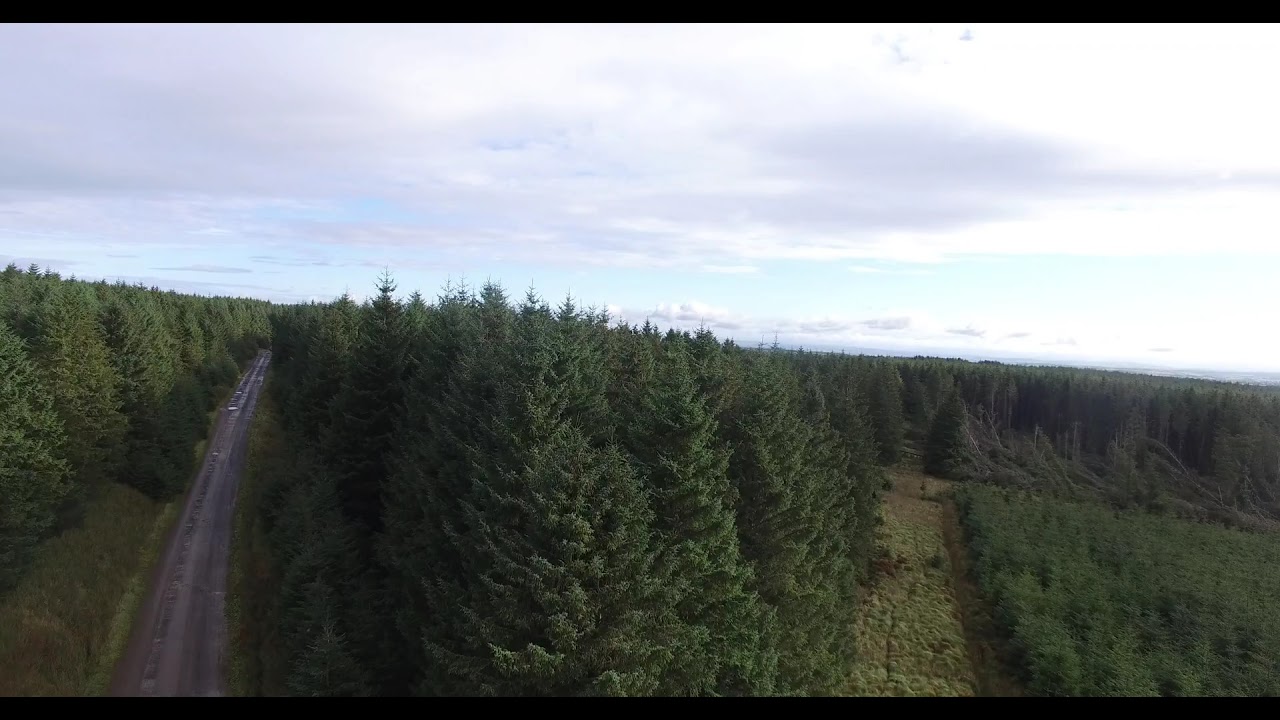This rectangular photograph, flanked by thin black letterbox bars at the top and bottom, offers a bird's-eye view of a serene, rural landscape dominated by deep green coniferous forests and a quiet country road. The road stretches diagonally from the bottom left to the middle of the image, seemingly paved yet worn with grooves, possibly indicating a mix of dirt and other materials. It's a two-lane stretch, bordered by tall, dense evergreen trees that create a canopy above and extend far into the distance. The trees on the left of the road form a dense forest, while on the right, a distinctive cleared area marks a tree farm with smaller evergreen trees planted in neat, orderly rows.

The tree farm transitions into a marshy, light-green clearing interspersed with felled trees, adding to the rustic atmosphere. The sky above is a pale blue, interspersed with thin, light gray clouds, casting a soft light over the entire scene. In the background, both sides of the road are framed by towering evergreen forests, enhancing the sense of isolation and natural beauty. Though vehicles are mentioned, they remain indistinct or entirely absent, giving the road a solitary, untouched feel. This detailed interplay between the road, dense forests, and the organized tree farm creates a vivid tableau of rural tranquility and natural order.